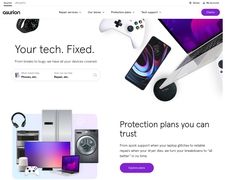This detailed infographic highlights various electronic devices and associated protection plans. The prominent text at the top reads "Your Tech," paired with an array of images to its right. These images include a white Sony PlayStation controller, a black cell phone, and a laptop displaying a dual-toned purple screen. Beneath this section, additional electronics are featured to the left of a square box, under which the text reads "Protection Plans You Can Trust." Further descriptions are provided below, adjacent to a prominent purple button. Among the displayed devices on the left side of the box are headphones, a flat-screen TV, a laptop, a washer and dryer, a refrigerator, and prominently in the forefront, another PlayStation controller.